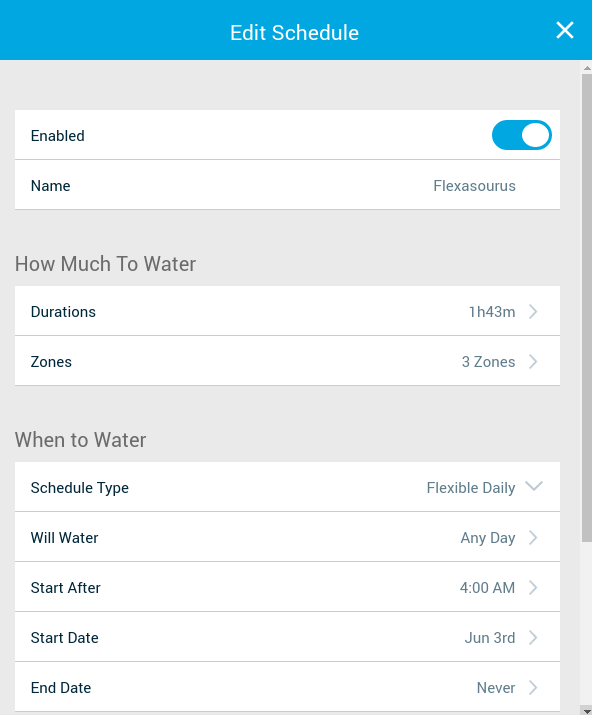**Detailed Caption:**

The image appears to be a screenshot from a website, showcasing a pop-up scheduling interface. The pop-up features a prominent blue header at the top, displaying the schedule title in white text, accompanied by a close button (marked with an 'X') in the right-hand corner. The main content of the pop-up is set against a grey background, and it includes various white information tables with black text. 

At the top of the content area, there's an 'Enabled' option with a blue slider that is toggled on. Below this, the name 'Flexasaurus' is listed, which likely serves as a nickname for a specific watering schedule or system.

The schedule details included are as follows:

- **Watering Duration**: 1 hour and 43 minutes
- **Zones**: 3 zones
- **Watering Frequency**: Any day
- **Start Time**: After 4 AM
- **Start Date**: June 3rd
- **End Date**: Never (ongoing)

A grey scrollbar is visible on the right side, indicating that more information is available beyond the visible portion of the pop-up. The darker portion of the scroll bar extends more than three quarters of the way down the screen, suggesting there may not be much more text below the current view.

The detailed schedule appears to be for a watering system, although the exact meaning of 'Flexasaurus' and the significance of the zones are not clearly explained. The long duration of 1 hour and 43 minutes for watering indicates a potentially extensive watering session, possibly managed by an automated sprinkler system.